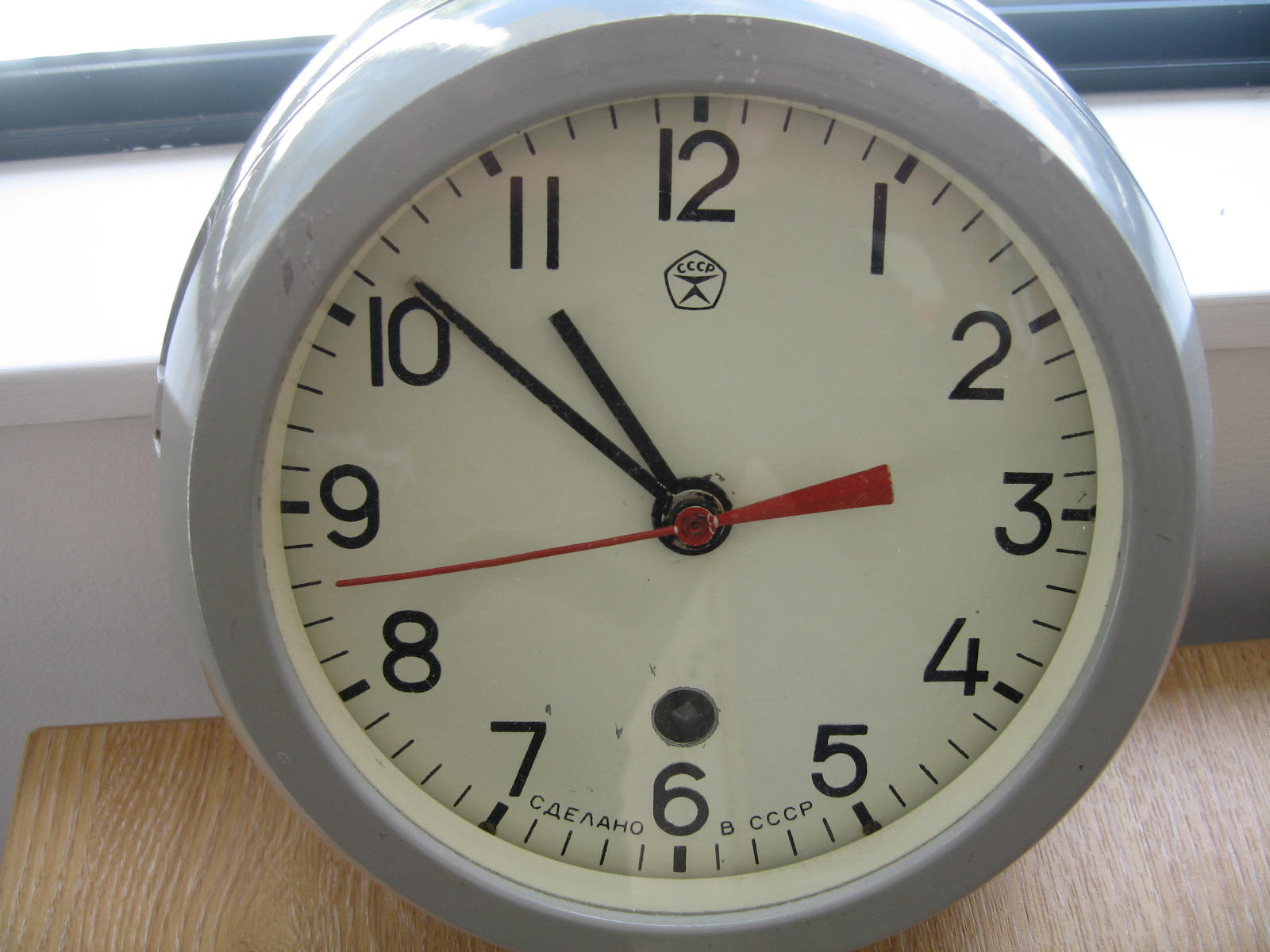This photograph captures a vintage-looking, large analog wall clock with a gray bezel showing slight scratches, leaning against the white, stone-like windowsill of a window with dark trim. The clock features a white face with black minute markers, a red second hand, and black hour and minute hands, indicating a time of approximately 10:52. The clock displays the text "CCCP" and additional Russian writing near the number 6, just above a keyhole for its mechanical winding mechanism. The setup suggests the clock is resting on a synthetic wood grain surface under daylight streaming through the window.